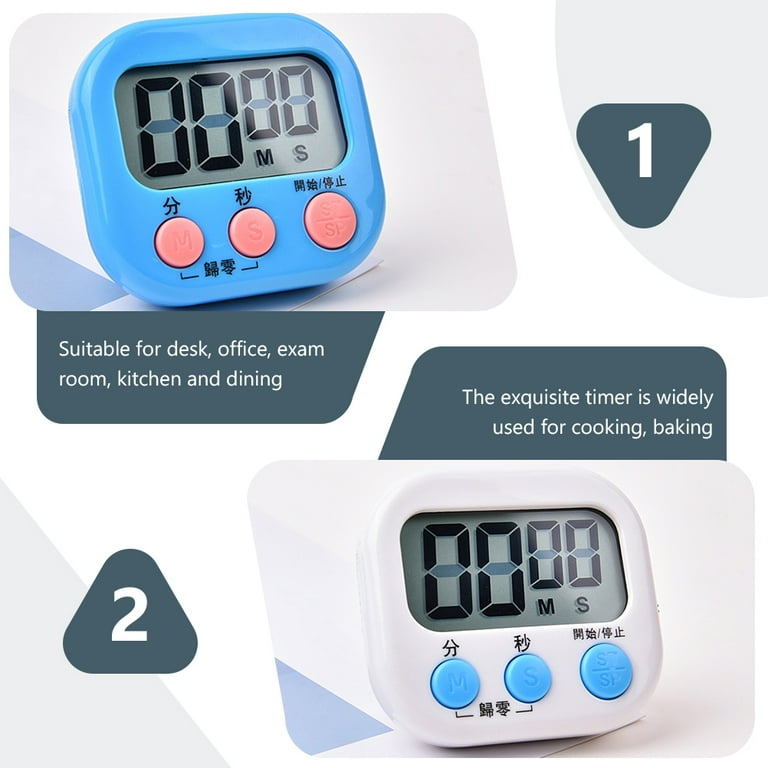This image is a detailed advertisement for a pair of small digital desk timers, emphasizing their suitability for a variety of uses. The timers are presented within a white and gray background. The upper timer, labeled with a rounded triangle marked "1", features a blue exterior with pink or salmon-colored buttons. The lower timer, marked with a similar but inverted triangle labeled "2", has a white cover with light blue buttons. Both timers have the same button arrangement and digital display: two large numbers at the center, flanked by two smaller numbers above which are the letters M and S. The M and S are also present on the physical buttons. The third button bears an "S over SI" with a minus sign. Chinese characters are prominently displayed above and below the buttons, indicating the product might be marketed in a Chinese-speaking region, though English letters are also used for the main functionalities.

Text in the middle of the image highlights the timers' versatility, with phrases like "suitable for desk, office, exam room, kitchen, and dining" and "the exquisite timer is widely used for cooking, baking." Despite slight differences in color, both timers share identical features, underlining their multi-purpose utility in various settings.